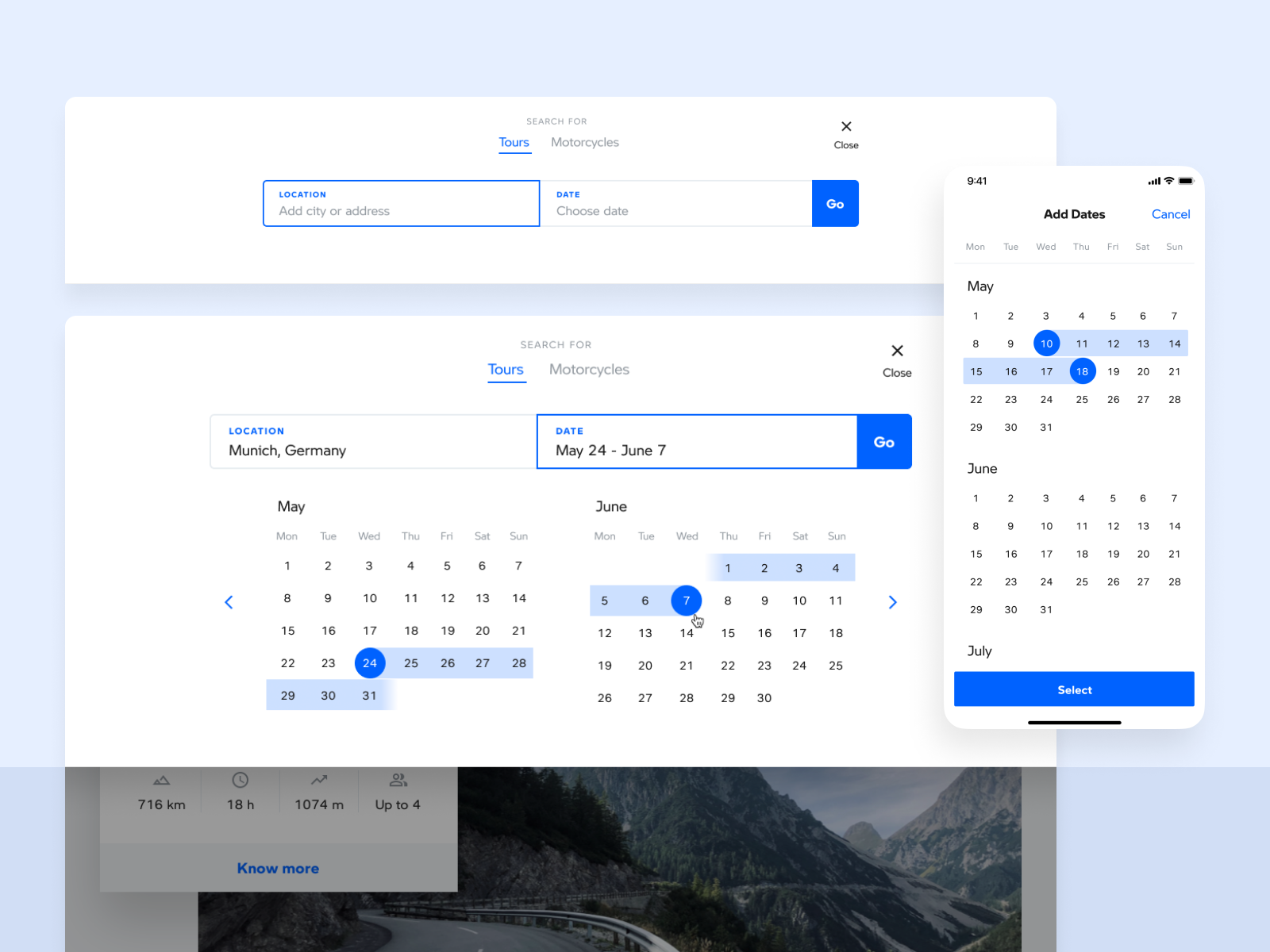The image features a detailed interface for selecting tour dates. The primary elements are as follows:

1. **Central Interface**: 
    - **Location Selection**: A white rectangle with a blue outline that prominently displays "Location" in blue text.
    - **Tour Information**: Above the location area, there's a central section with black text and a prominent "Tours" in blue, underlined. There is a gray word near this, though it's unclear.
    - **Date Selection**: A gray outlined rectangle labeled "Date," with "Choose Date" written beneath it.
    - **Action Button**: A blue square that reads "Go" in white text.

2. **Detail Box**: 
    - **Tour Modal**: Below the main interface lies an additional white rectangle detailing "Tours" (underlined) and another word starting with "Motor," but further text is unclear.
    - **Close Button**: An "X" with "Close" beneath it.
    - **Location Details**: A gray rectangle stating "Location" in blue, followed by "Munich, Germany."
    - **Date Range**: A blue outlined rectangle with the dates "May 24th through June 7th."
    - **Action Button**: Another blue square bearing the text "Go."
    - **Calendars**: 
        - **May and June Calendars**: Feature a start date circled in blue, with subsequent dates shaded in blue.
        - **June Calendar**: Features the last date circled in blue with previous dates shaded similarly.

3. **Additional Control Panel**: 
    - Overlapping the central interface is another white rectangle with partially visible text.
    - **Options Available**: 
        - "Add Dates" is centered in black.
        - "Cancel" appears to the right.
    - **Calendars for Selection**:
        - **May Calendar**: Some dates circled in blue, lighter blue filled squares, and a longer blue rectangle labeled "Select."
    - **June Calendar**: Similar to the May Calendar in functionality.

4. **Background Image**: 
    - **Scenic Element**: Partially visible at the bottom, depicting what appears to be a mountain landscape, though obscured by the interface elements.

The overall layout and design provide an interactive experience for users to select their desired tour dates and other relevant logistics, framed in a user-friendly blue and white color scheme.